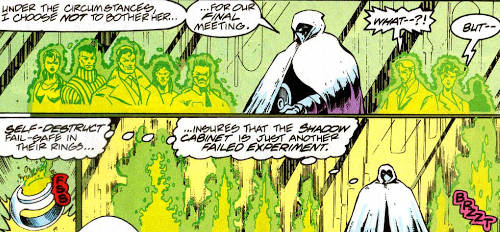The image is a brightly colored comic book page featuring two distinct scenes, top and bottom. In the top panel, which stretches across the page, a character stands center stage in a striking outfit consisting of a white cloak, a white mask edged with black, and a black stomach area. Surrounding this central figure are five glowing green figures to the left and two to the right. The background features clear windows with white and black diagonal stripes. The central character declares, "Under the circumstances, I choose not to bother her for our final meeting." One of the characters on the right responds with "What?" while another attempts to interject with "but."

The bottom panel features a close-up of a detonating device emitting white, silver, and green hues, with red text exclaiming "FBS." This scene also includes a zoomed-in section from the top panel, now showing four glowing figures on the right and one on the left, amidst a backdrop of green fire with the black text "BRZZT" outlined in purple. The cloaked character, looking directly at the audience, ominously states, "Self-destruction fail-safe in their rings ensures that the Shadow Cabinet is just another failed experiment."